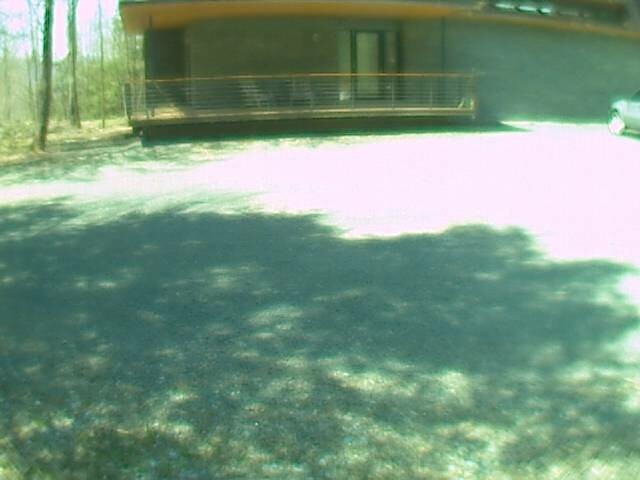This outdoor photograph captures a quaint, single-story house under a blue sky with scattered white clouds. Dominating the foreground is a grassy area mixed with pebbles and small rocks, suggesting a rustic parking lot. The sunlight streaming in from the right side creates bright, blown-out spots on the ground. To the right of the house, a partially visible car is parked in front of a cinder block or brick wall. The house, possibly made of stone, features a wraparound porch enclosed by a low fence. On the porch, there are two chairs beside a glass door. Extending from the porch is a covered area supported by the roofline. Surrounding the house on the left are trees, some with sparse foliage, contributing to a natural, slightly wild look. Shadows of the trees above cast intricate patterns of light and shade across the bottom two-thirds of the image, adding depth and contrast.